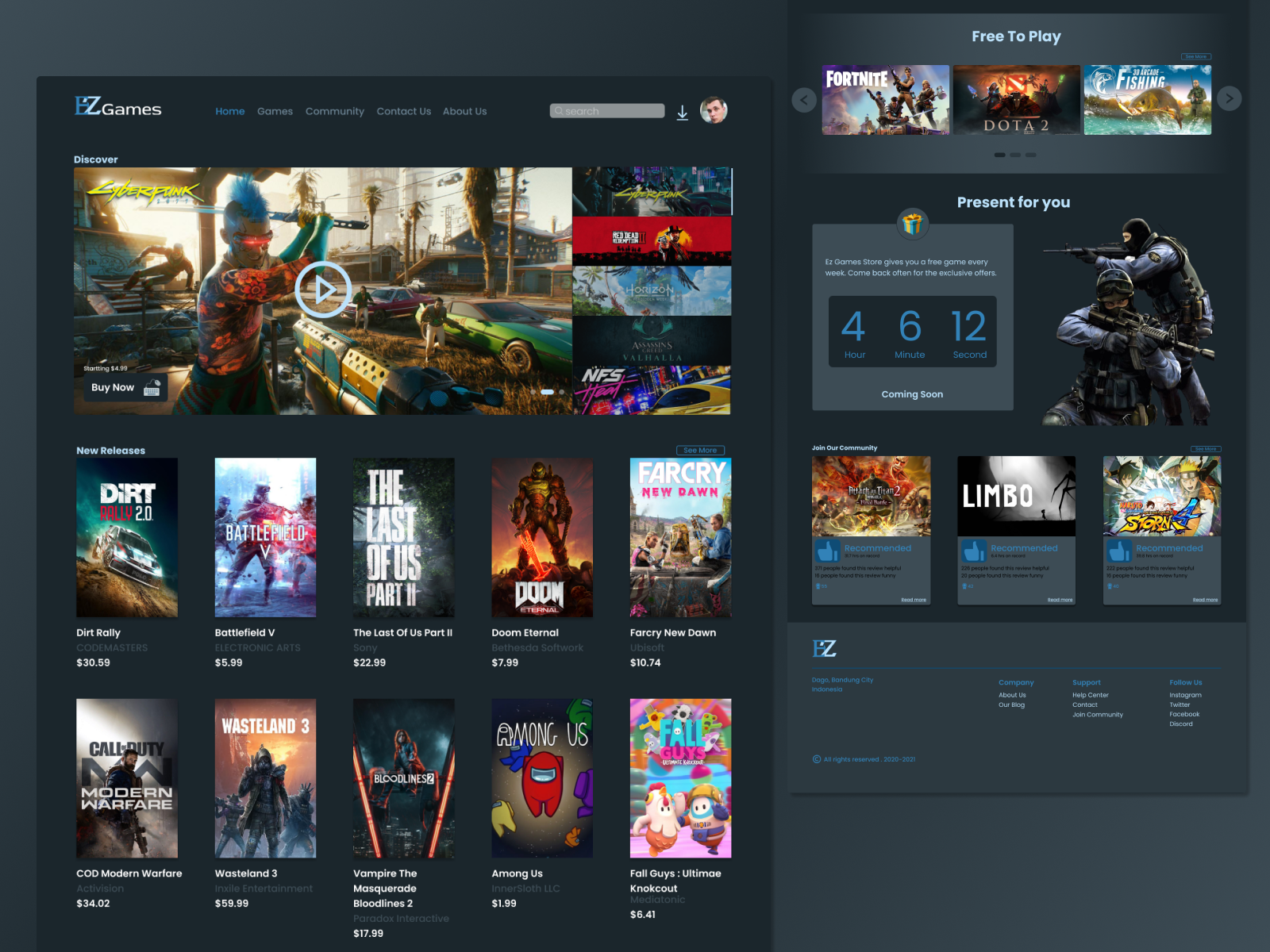The image depicts the digital storefront of a gaming client named 'Easy Games,' which closely resembles popular platforms like Steam. The interface showcases a variety of tabs at the top, including Home, Games, Community, Contact Us, and About Us. The user is currently on the homepage, which prominently features a range of purchasable games such as "Dirt Rally 2," "Doom Eternal," "Battlefield 5," and "The Last of Us Part 2." Many of these titles are listed at significantly reduced prices, indicating ongoing sales or that the games have been available for an extended period. On the right side of the screen, there's an attention-grabbing countdown timer for the upcoming release of a new Call of Duty game. Additionally, a banner at the top highlights a free-to-play section, featuring popular games like "Fortnite," "Dota," and a fishing game. The overall layout is designed to facilitate easy navigation and quick access to various gaming options.